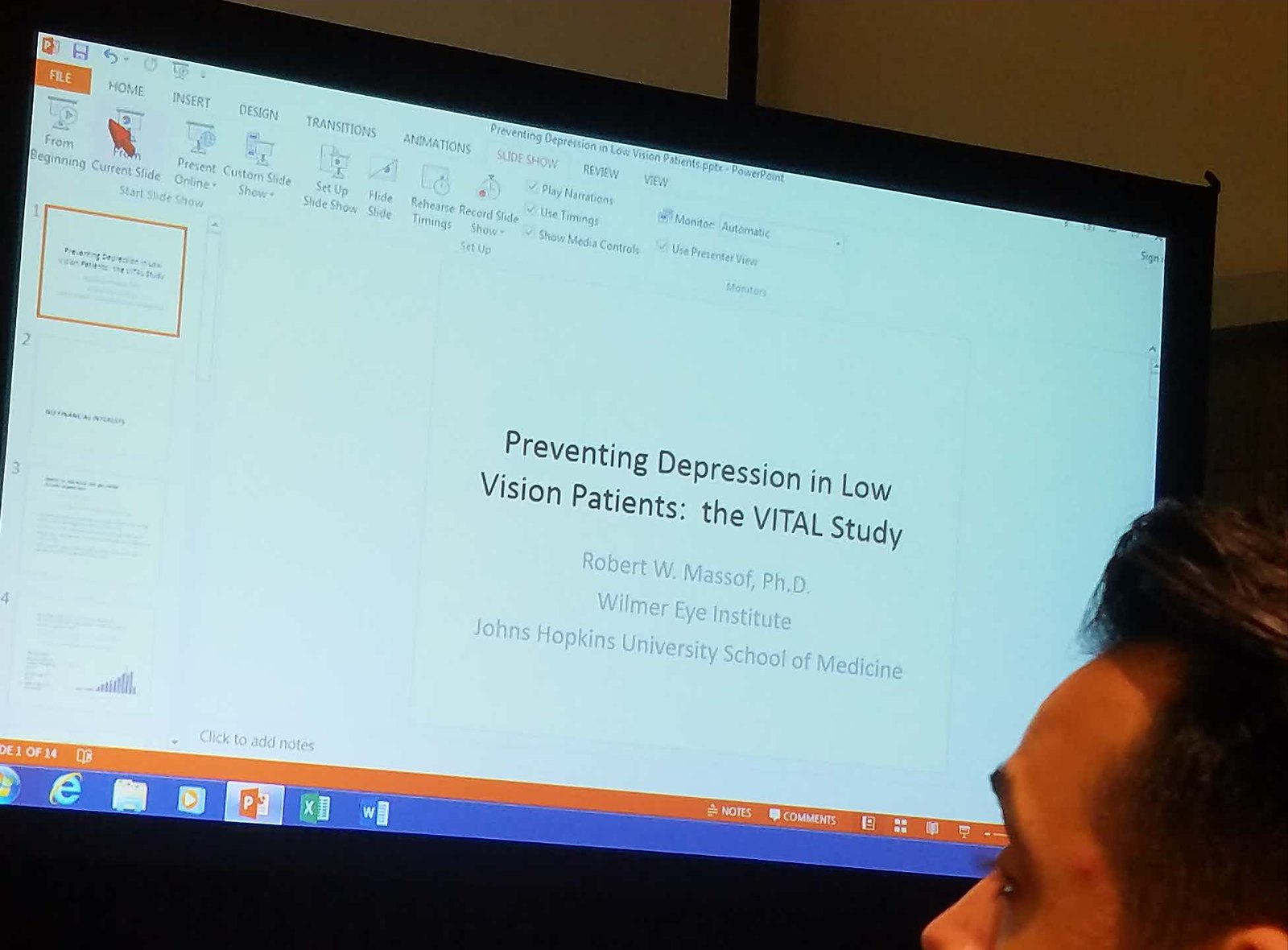This horizontal rectangular image depicts a computer screen mounted at eye level, seen from a standing person's perspective. In the lower right corner is a partial view of a man's head with brown hair, styled with more volume on top and shaved on the sides. His eyes are directed at the screen, which displays a PowerPoint presentation. The title at the top reads "Preventing Depression in Low Vision Patients.PPTX PowerPoint." The screen is predominantly white with a black border, and the toolbar at the top showcases various tabs including File, Home, Insert, Design, Transitions, Animations, Slide Show, Review, and View. The main slide in the center bears the title in black text: "Preventing Depression in Low Vision Patients: The Vital Study." Below this, the presentation credits Robert W. Massoff, Ph.D., from the Wilmer Eye Institute, Johns Hopkins University School of Medicine.